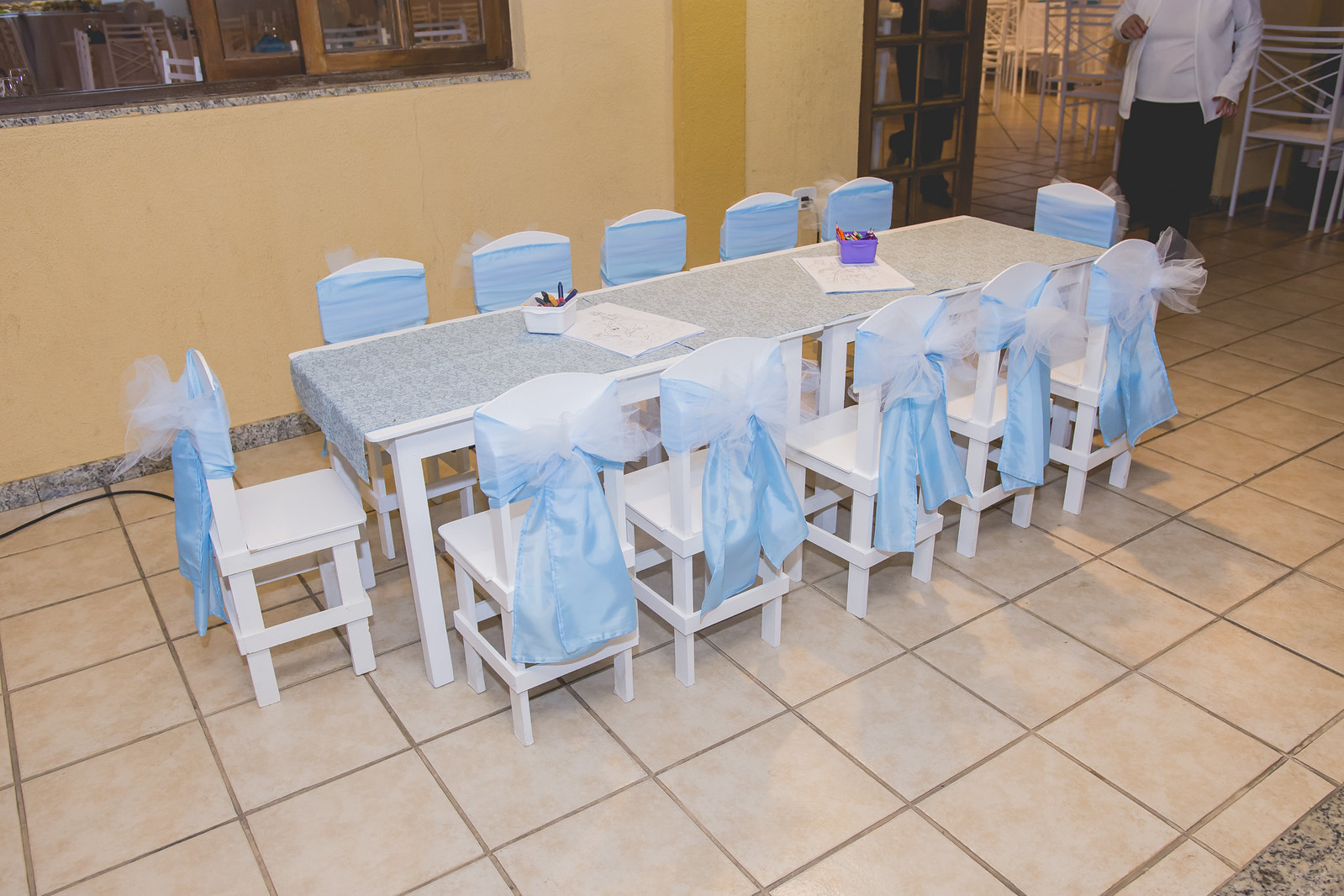The image showcases an elegantly arranged table setting likely situated inside a restaurant, suggested by the beige-ish tiled floor and peach-colored walls. The primary focus is a long, narrow white table adorned with a tablecloth runner. Surrounding the table are white wooden chairs, each detailed with a large satin blue bow tied around the back, overlaid with a delicate, see-through white netting. The arrangement includes ten chairs on each side and one chair at each end, making a total of twelve. The table, set lower to the ground, appears designed for children, possibly for a kid's party. Items like paper and crayons are scattered on the table, reinforcing the child-friendly theme. In the background, a section of the restaurant with tall chairs is visible, alongside a cutout window on a yellow-orange wall, adding to the ambiance. A person dressed in black pants, a white shirt, and a white jacket stands nearby.